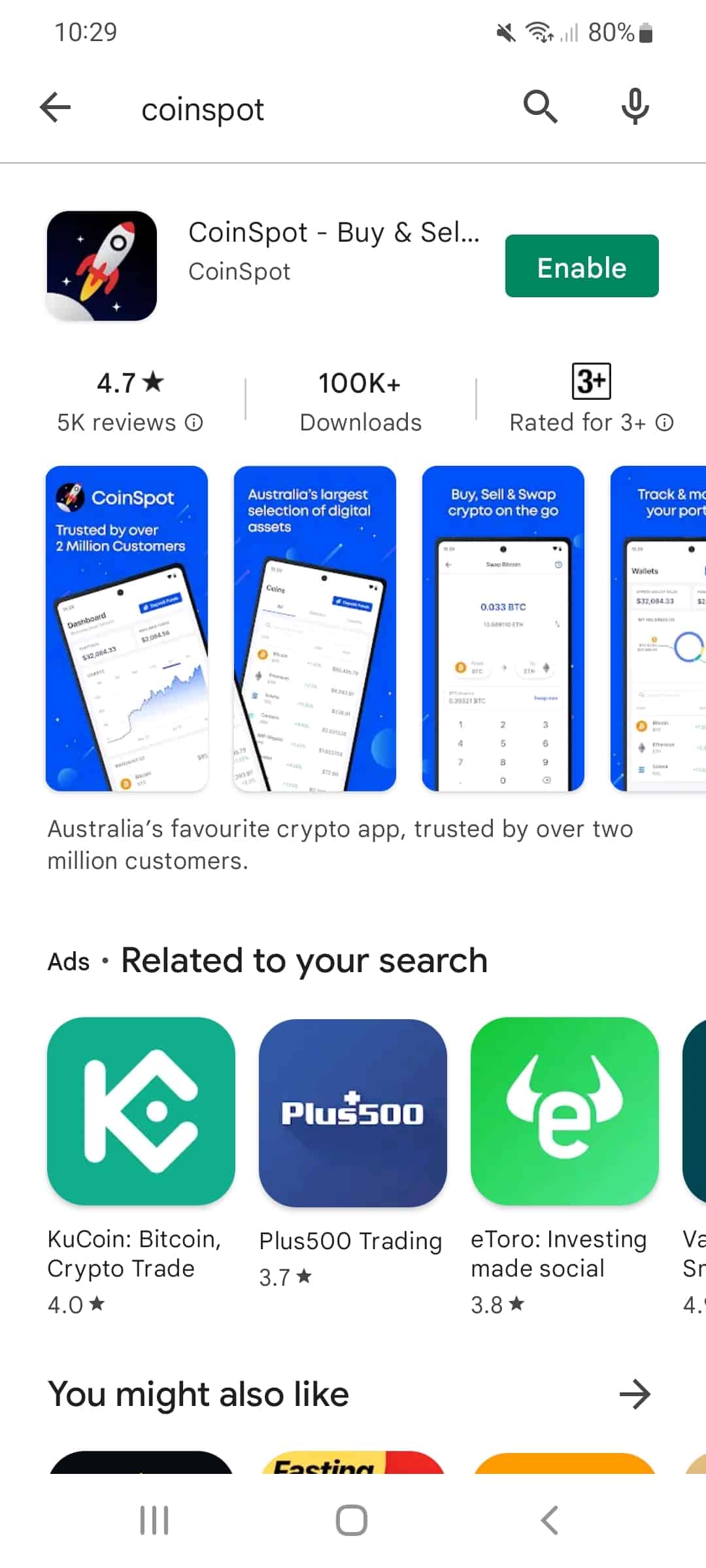**Screenshot of a Coinspot Search on a Smartphone**

The image shows a smartphone screen capturing a search query for "Coinspot." At the very top, the time is displayed as 10:29 in the top left corner, accompanied by a muted sound icon, a strong Wi-Fi signal, a full bars indicator, an 80% battery charge, and the corresponding battery icon.

Below this status bar, a light gray line spans horizontally across the screen, demarcating the search bar area. The search bar starts with a left-pointing directional arrow, then the word "Coinspot," followed by a magnifying glass icon, and a microphone icon.

Underneath the search bar, a dark gray, rounded-corner square appears against a white background, decorated with small white stars, a moon at the edge, and a gray and red rocket ship. Next to this icon, bold text reads "Coinspot, buy and sell," with a subtitle of "Coinspot" followed by a button labeled "Enable."

The next section features user engagement statistics: "4.75k reviews," indicating positive feedback, "100k downloads," and a "3+ rating," suitable for ages three and up.

Prominent below this are four vertical rectangular cards filled with dark blue backgrounds, each displaying a screenshot from the Coinspot app.

Following the visuals, there is a text in black stating, "Australia's favorite crypto app trusted by over 2 million customers."

Afterward, the section labeled "Ads related to your search" is presented, listing three additional apps: "KuCoin - Bitcoin Crypto Trade 4.0," "Plus 500 Trading 3.7 stars," and "eToro - Investing Made Social 3.8 stars."

Finally, a prompt at the bottom reads "You might also like" with a right-pointing directional arrow, suggesting more options.